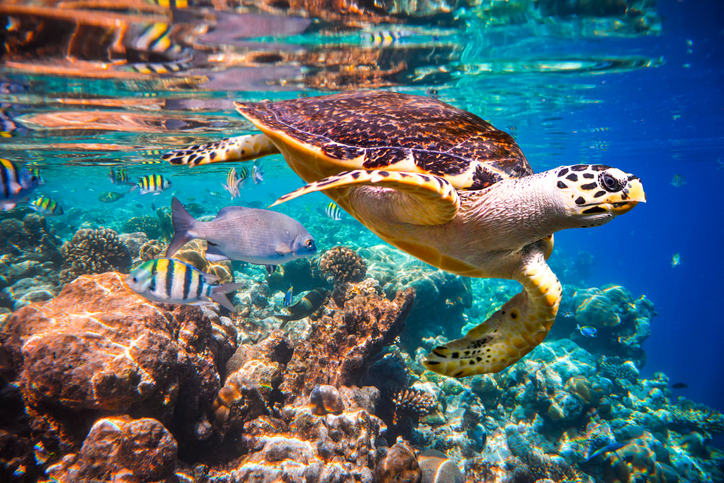An exquisite underwater photograph captures a large turtle swimming centrally beneath the blue ocean surface. The turtle’s beige body, with a yellowish tint on its legs, features a brown-spotted head and a striking yellow beak. The turtle's brown shell, accented with lighter and orange tones, contrasts beautifully with its surroundings. The photo also reveals a vibrant underwater ecosystem, including submerged boulders, coral reefs, and a variety of fish - some with black stripes and yellow hues, others in gray - swimming around. Ripples at the top of the image hint at the turtle's recent dive, adding a dynamic element to this captivating marine scene.